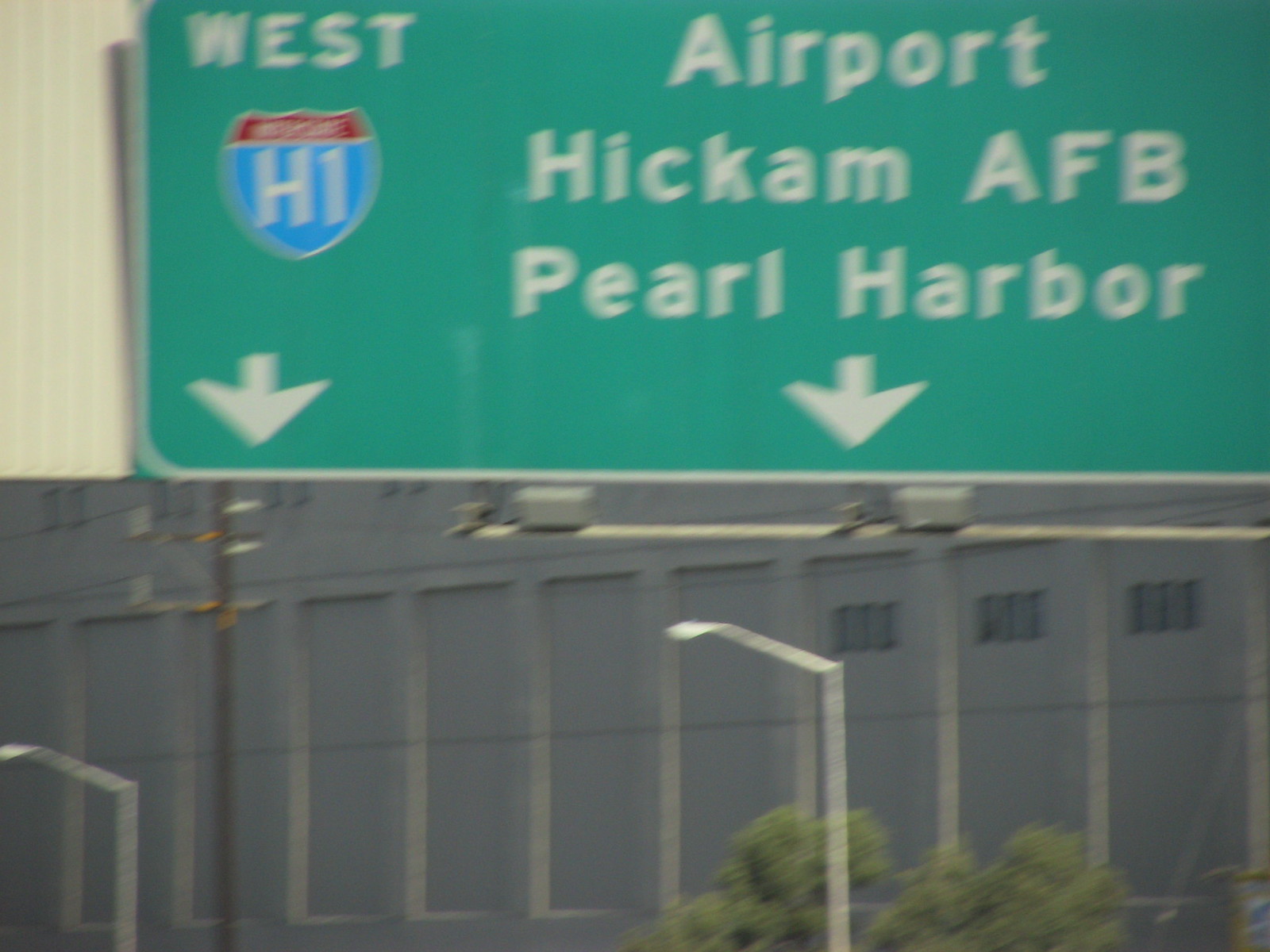This photo, though somewhat blurry, captures an urban scene featuring various elements. Dominating the bottom portion of the image is a dark gray building, partially obscured by the green tops of two trees. In the foreground, two street lights rise up, accompanied by the back of a traffic light and an electrical pole with wires stretching across the top of the frame.

Positioned prominently towards the top is a street sign with a green background and predominantly white lettering. The sign reads "West" and features a shield emblem, colored red on the top half and blue on the bottom, inscribed with "HI" or "H1" in white on the blue portion. Below this emblem is a downward-facing arrow. The rest of the sign directs drivers to three locations with another downward arrow: Airport, Hickam AFB, and Pearl Harbor.